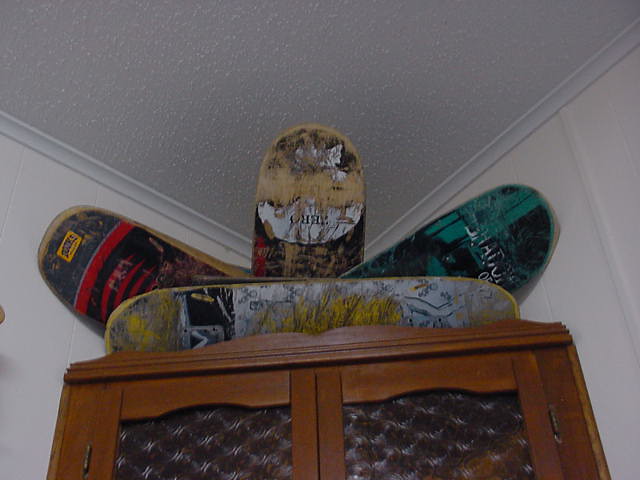The interior of a home is showcased in this color photograph, featuring the top section of a dark brown, antique wooden china cabinet. The visible portion of the cabinet, which occupies the bottom third of the image, includes doors fitted with intricately scalloped, thick, coke-bottle glass that obscures the contents within. Resting atop the cabinet is a curated display of four weathered and heavily used skateboard decks, notable for their lack of wheels. Two of the skateboards are angled to the sides, one points straight up, and the fourth lies flat at the bottom, partially visible. The decks, whose underlying wood peeks through worn paint, sport an array of colors: green and black, red and black, yellow and white, and one so extensively worn that only white remnants remain visible. The white wall behind them, with its trim and dated popcorn ceiling, provides a stark contrast, highlighting the skateboards' vibrant, hand-painted designs.